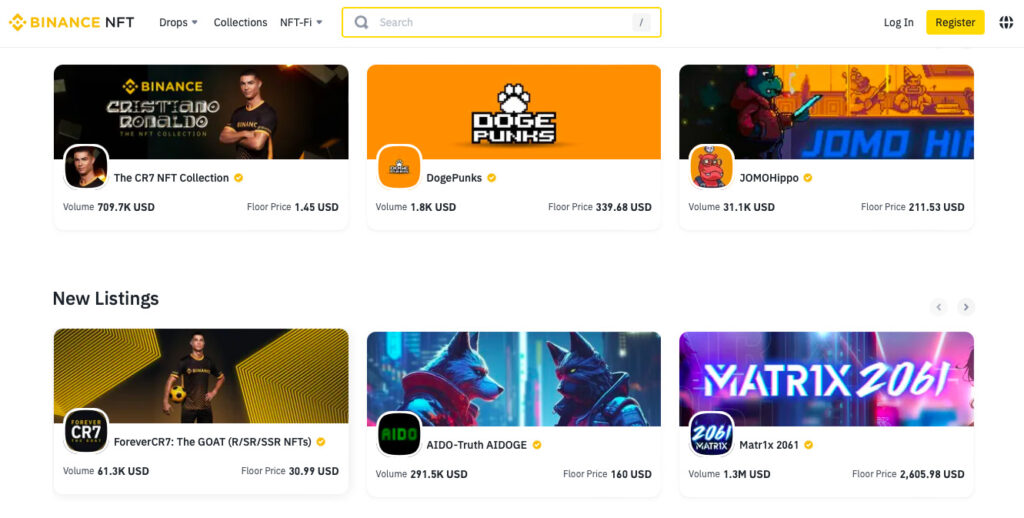The image depicts the homepage of Binance NFT, showcasing various curated collections of digital artwork and their respective market values. Prominently featured is the "CR7 NFT Collection," which boasts a total estimated value of $709.7 thousand. Adjacent to it is "Doge Punks," valued at $1.8 thousand. Another notable collection is "Jomo Hippo," with a valuation of $31.1 thousand. Below these, the "ForeverCR7, the GOAT" collection is displayed, listing S, SR, and SSR NFTs, collectively worth $61.3 thousand. The "IDO Truth" (IDOJ) collection appears next, with an impressive total of $291.5 thousand. Dominating the chart is "Matrix2061" (styled as M-A-T-R-1-X), with an astounding valuation of $1.3 million, making it the most valuable collection on display.